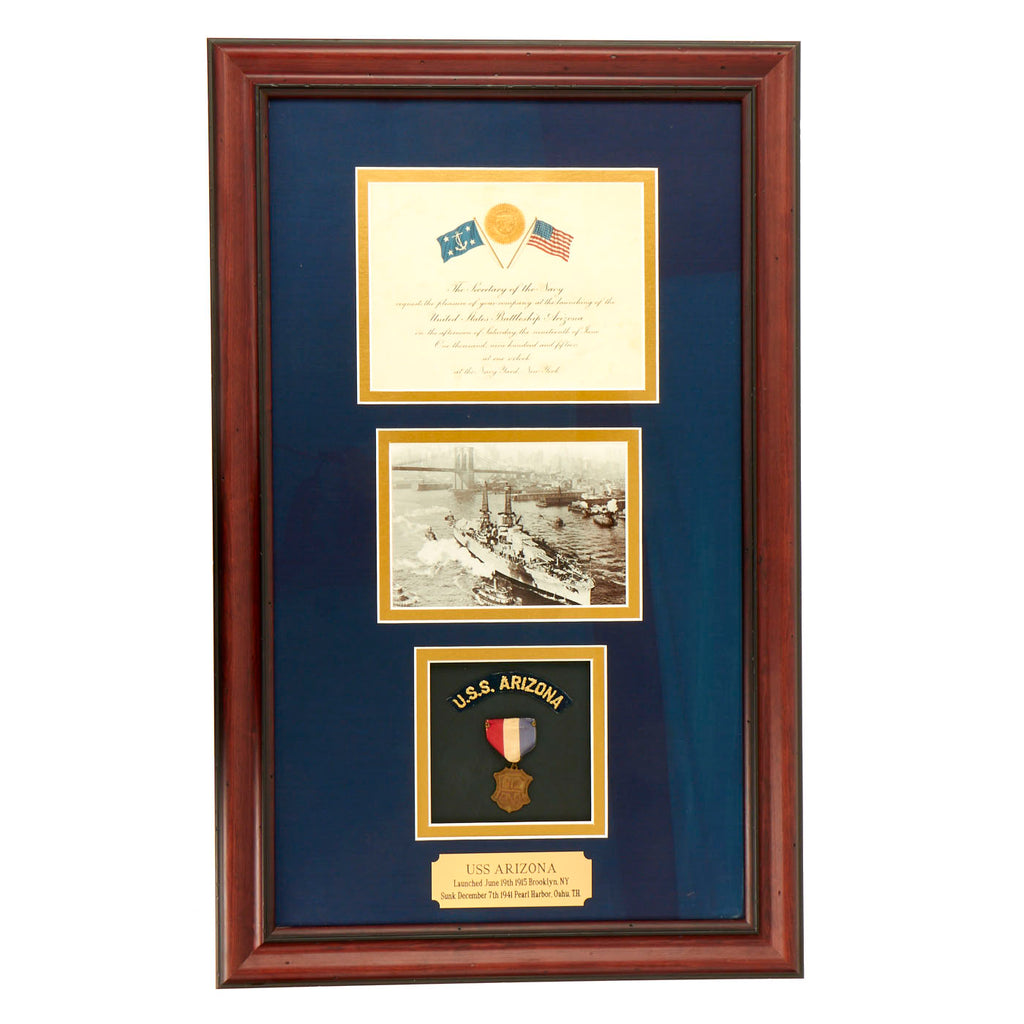This is a detailed image of a commemorative plaque honoring the USS Arizona. The plaque is housed in a mahogany frame and features a dark blue backing. The centerpiece at the bottom showcases a gold plate that reads "USS Arizona," though only "Brooklyn, New York" is clearly legible on it. Above the plate is an image of the USS Arizona itself, bordered by a yellow-orange square.

The plaque is designed with layered sections: directly above the gold plate is another section that says "USS Arizona," bordered identically in yellow-orange. An image of the ship occupies a rectangular space above, with the same border style. Topping the layout is a document prominently displayed, featuring the American flag and a seal in the middle. The document also shows a blue flag with an anchor on it to the left, surrounded by ornate calligraphy that remains unreadable.

The meticulous arrangement and design details of the plaque serve as a respectful tribute to the historical significance of the USS Arizona.